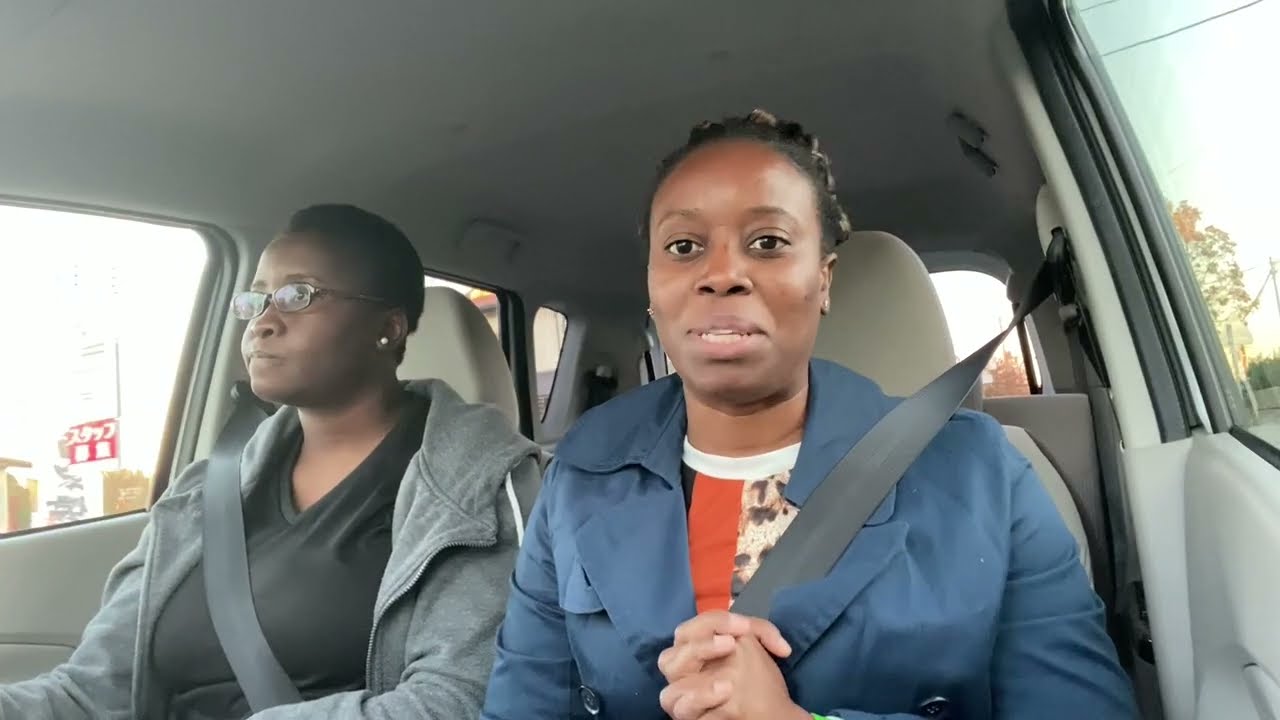In a horizontally aligned rectangular image, the scene is set inside a car with a distinctly gray interior, including the ceiling, seats, and door panels. Two African-American women, evidently comfortable and friendly with each other, occupy the front seats, both secured with gray seatbelts. The woman in the driver's seat on the left is gazing to the left side of the image. She has dark skin, short black hair, and wears glasses and stud earrings. Her attire includes a V-neck dark gray T-shirt underneath an unzipped gray hoodie-style jacket. The passenger, seated on the right, with slightly up-braided hair, observes the road ahead, sharing a subtle smile that reveals some of her teeth. She is clad in a blue coat over a multicolored shirt with a prominent orange stripe and a white crew neck collar and also wears earrings. Her hands are folded casually in front of her. Outside the car's windows, a hint of the environment can be seen, including some trees, power lines, and a red sign, indicating it is daytime.